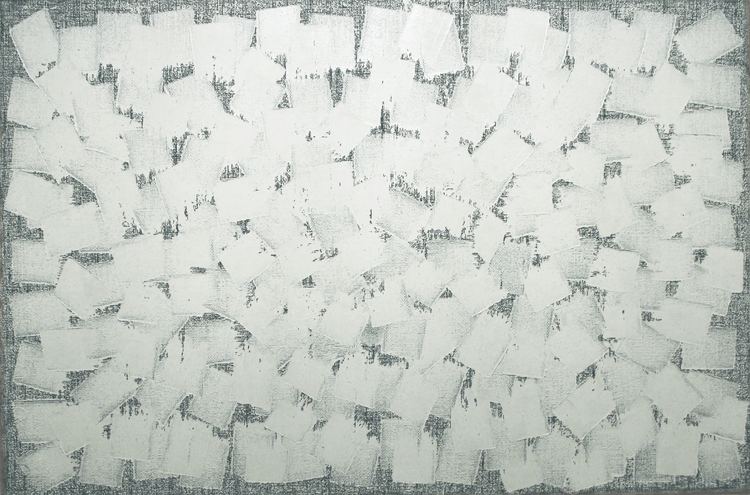This image depicts an abstract, modern painting with a prominent geometric theme. The background is a noisy gray color, accentuated by the visible texture and threads of the canvas poking through. In the foreground, approximately 100 white rectangular shapes, resembling sheets of paper, are layered and overlapping, creating a three-dimensional effect. The white rectangles vary in shape; some have straight edges while others feature irregular, drippy edges. The rectangles are brighter compared to the gray background, enhancing the depth and layering effect. The overall composition forms a cohesive rectangular mass of these overlapping shapes, arranged in a pattern that repeats over and over with subtle variations, giving the image a dynamic yet uniform appearance.